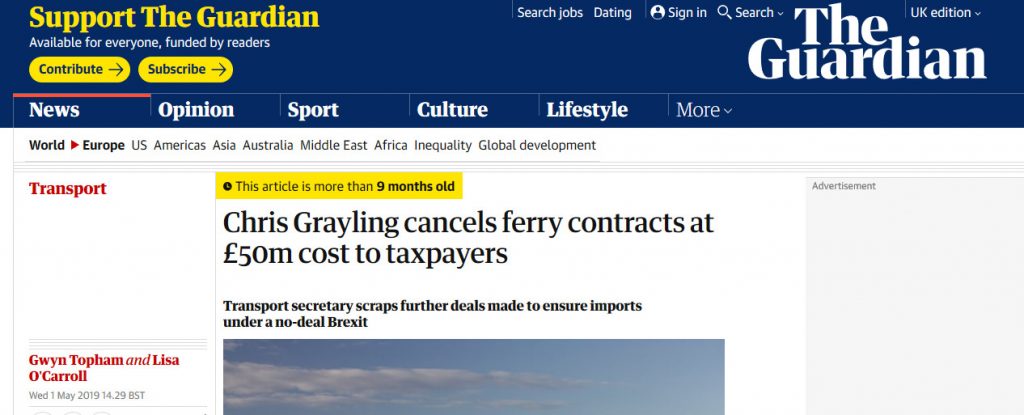The image is a screenshot of a webpage from The Guardian, a well-known British newspaper. At the top left corner, there is a yellow call-to-action text that reads, "Support The Guardian," followed by a smaller, white text stating, "Available for Everyone, Funded by Readers." Directly beneath, two boxes are visible: the left one labeled "Contribute" with a rightward arrow, and the right one labeled "Subscribe," also accompanied by a rightward arrow.

On the top right of the image, "UK Edition" is displayed along with a drop-down arrow. Centrally placed at the top, "The Guardian" is prominently featured in bold white letters. Below this, the navigation bar presents additional categories: "Search Jobs," "Dating," "Sign In," and a search icon.

Further down, there are six primary navigation categories starting from the left: "News," "Opinion," "Sport," "Culture," "Lifestyle," and "More," with "More" having an adjacent drop-down arrow.

In the middle of the image, an article headline captures attention: "Chris Grayling cancels ferry contracts at £50 million cost to taxpayer." Beneath this headline, a subheading provides more context: "Transport Secretary scraps further deals made to ensure imports under a no-deal Brexit."

This detailed depiction encapsulates both the navigational features of The Guardian's website and a specific news article being highlighted.